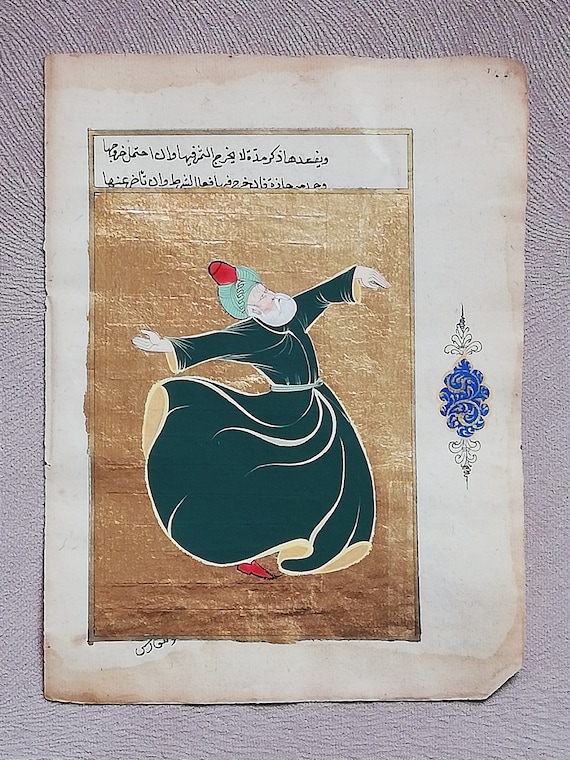The photograph, taken indoors, captures what appears to be an ancient, highly detailed Muslim painting on a yellowed piece of paper, possibly a page from a book. The paper is placed against a light mauve stucco wall. Central to the image is a depiction of an older man with light skin, a thick white beard, and mustache, who is likely a whirling dervish given his twirling posture. His head tilts back as he gazes upwards, arms dramatically extended with one palm facing down and the other up. He wears a dark green, floor-length tunic with a light green belt and gold undersides, accompanied by a single red shoe. Atop his head, he dons a light greenish-blue turban wrapped around a red fez. The painting's background is lavishly filled with gold leaf, creating a visually rich backdrop. Above the figure, there is black text in Arabic, and to the right is a floral emblem featuring a blue and gold leafy design with black embellishments. Notably, the paper shows signs of wear, including water damage at the top and bottom.